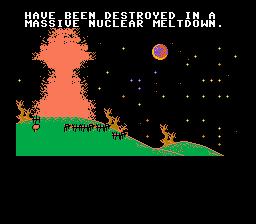The image appears to be a screenshot from a computer game. The background is entirely black, creating a stark contrast with the elements in the foreground. At the top of the image, text reads, "have been destroyed in a massive nuclear meltdown." 

Approximately a third of the way up from the bottom, a green rolling hill stretches across the scene, larger on the left side than on the right. The hill features simple, minimalistic drawings that resemble either people or fences, depicted as vertical black lines with horizontal lines intersecting them.

Atop the larger left-hand side of the hill, there's a depiction of a nuclear explosion. The explosion is illustrated with a light pink and peach smoky haze rising into the sky. The sky itself remains a deep black, dotted with small white stars and featuring a celestial body that seems to be the moon. This moon is distinctively embellished with hues of gold, purple, and pink, lending it an almost otherworldly appearance.